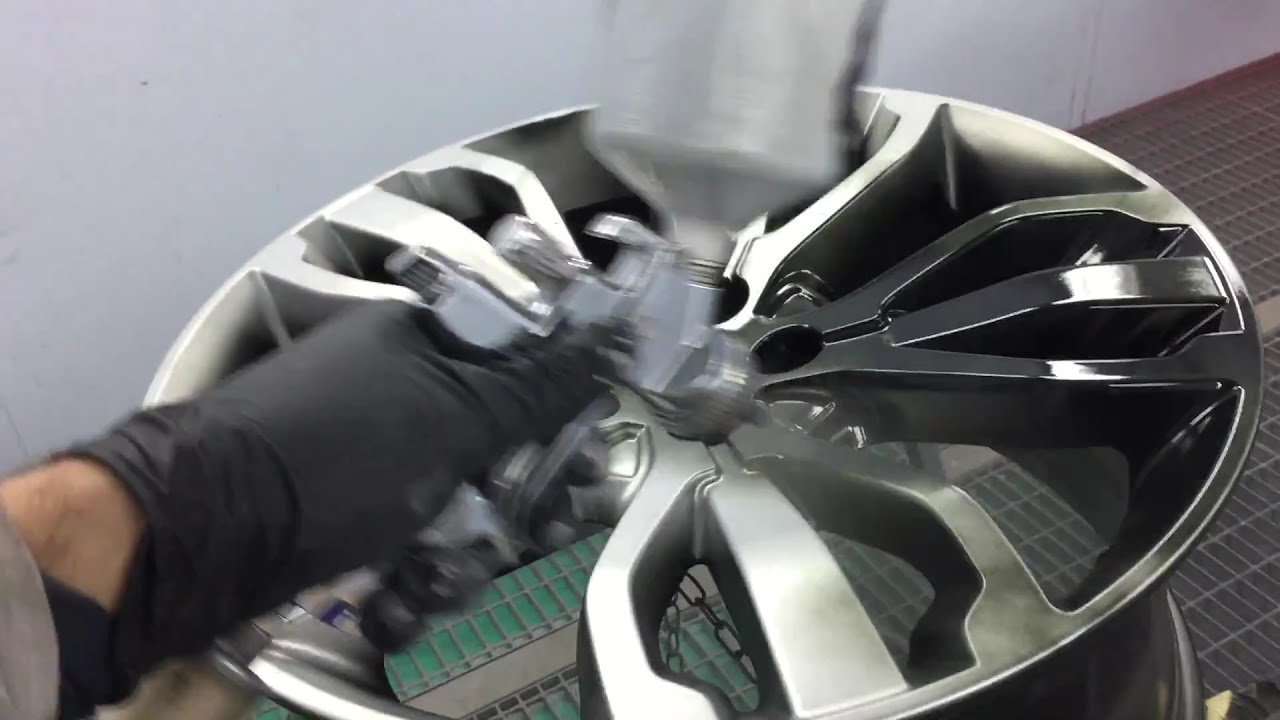A light-skinned person with hair on their arm, likely male, is meticulously spray-painting a chrome car wheel using black paint. The wheel, possibly a hubcap, features intricate designs with groups of three chrome columns radiating from the center. The person is wearing black latex work gloves, which are slightly wrinkled at the wrist, and the glove-clad hand is the focus at the lower left of the image. The individual is holding a spray paint can, positioned from the top center towards the hubcap, to ensure an even coat of black paint. The setting includes a metallic grated surface below the wheel to catch excess paint, with a predominantly gray and brownish-gray backdrop. The image, a rectangle almost twice as wide as it is tall, captures the meticulous process of transforming the wheel's appearance amidst a functional, industrial workspace.